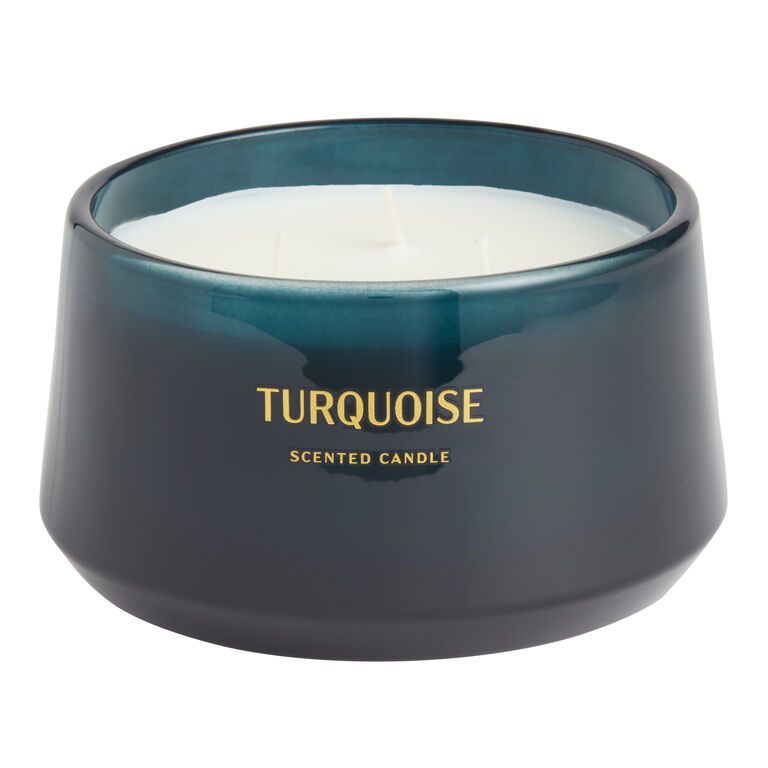On a pristine white surface, a sleek candle holder stands out prominently. The holder is a deep, dark turquoise color that almost appears black towards the bottom, transitioning to a semi-transparent teal near the top, allowing glimpses of the white wax inside. The bowl-shaped holder has a straight edge that tapers slightly upwards, lending it a modern and elegant profile. Printed in shiny gold letters on the side are the words "TURQUOISE" in large text followed by "scented candle" in smaller lettering underneath. The candle itself, a smooth flat mass of white wax, reveals three faintly visible wicks arranged in a triangular pattern at its center. The reflective quality of the holder captures the light beautifully, creating a striking contrast against the plain white background.